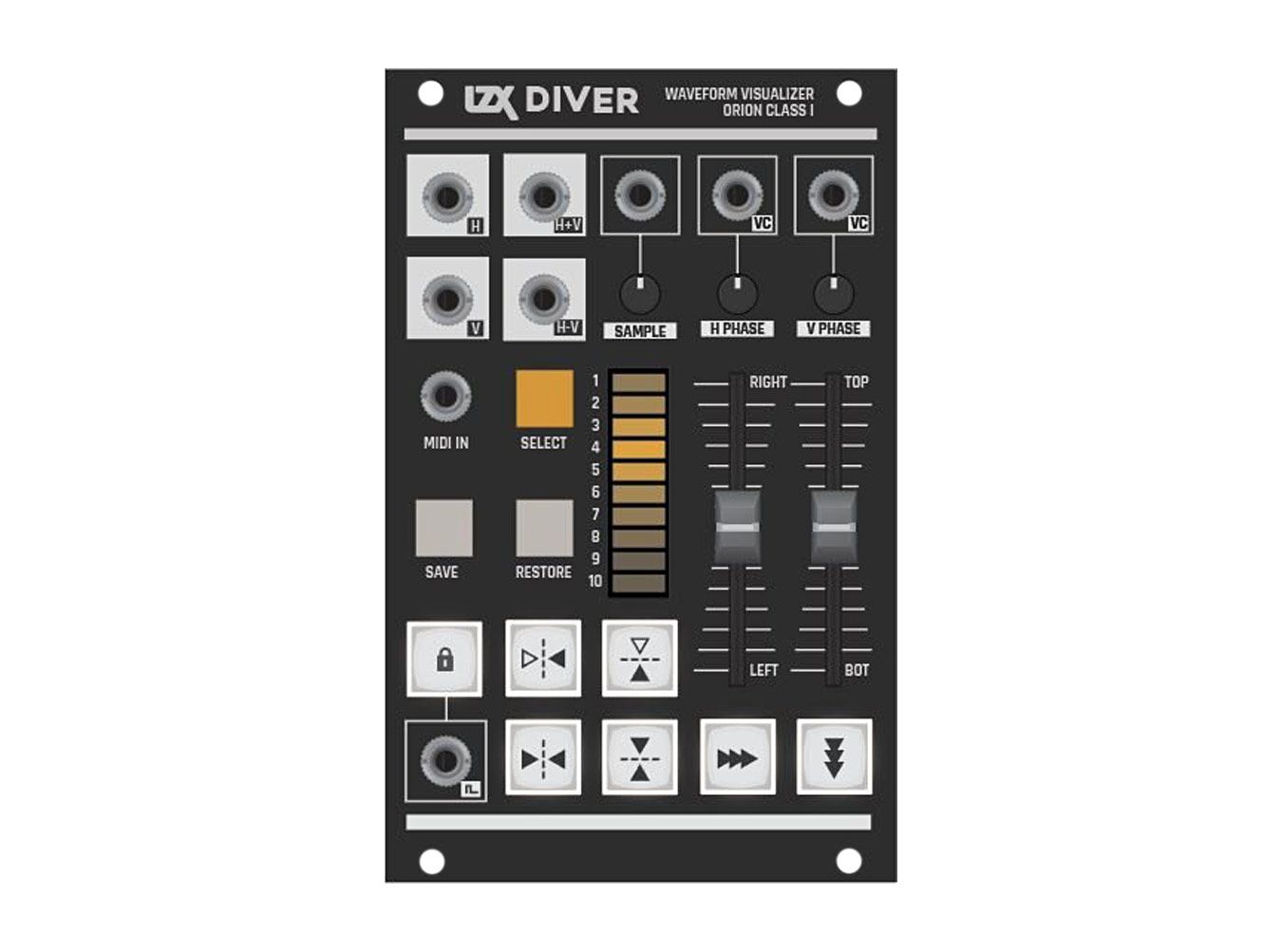The image is a detailed photograph of a rectangular electrical mixer device set against a white background. The device appears to be dark grey to black in color and features multiple lines of text, plugs, and dials, characteristic of audio or DJ equipment. The top of the device reads "LZX Diver, Waveform Visualizer Orion Class 1" in grey text, underscored by a thick grey line. Four silver plugs, each encased in grey squares, are visible beneath this line on the left. The device's faceplate has holes in all four corners, revealing the background. Seven knobs are spread across the middle section: the first two are housed in white squares with grey and black circles, while the next five are black squares with grey circles and black centers. Additional controls include fader knob buttons, dials labeled "right," "top," and "left," and buttons for "Select" (yellow), "Save," "Restore" (white), "Play," "Rewind," "Forward," and "Back," also in white with black lettering. At the bottom of the device are more plugs and a line, completing a sophisticated control interface designed for audio manipulation and visualization.